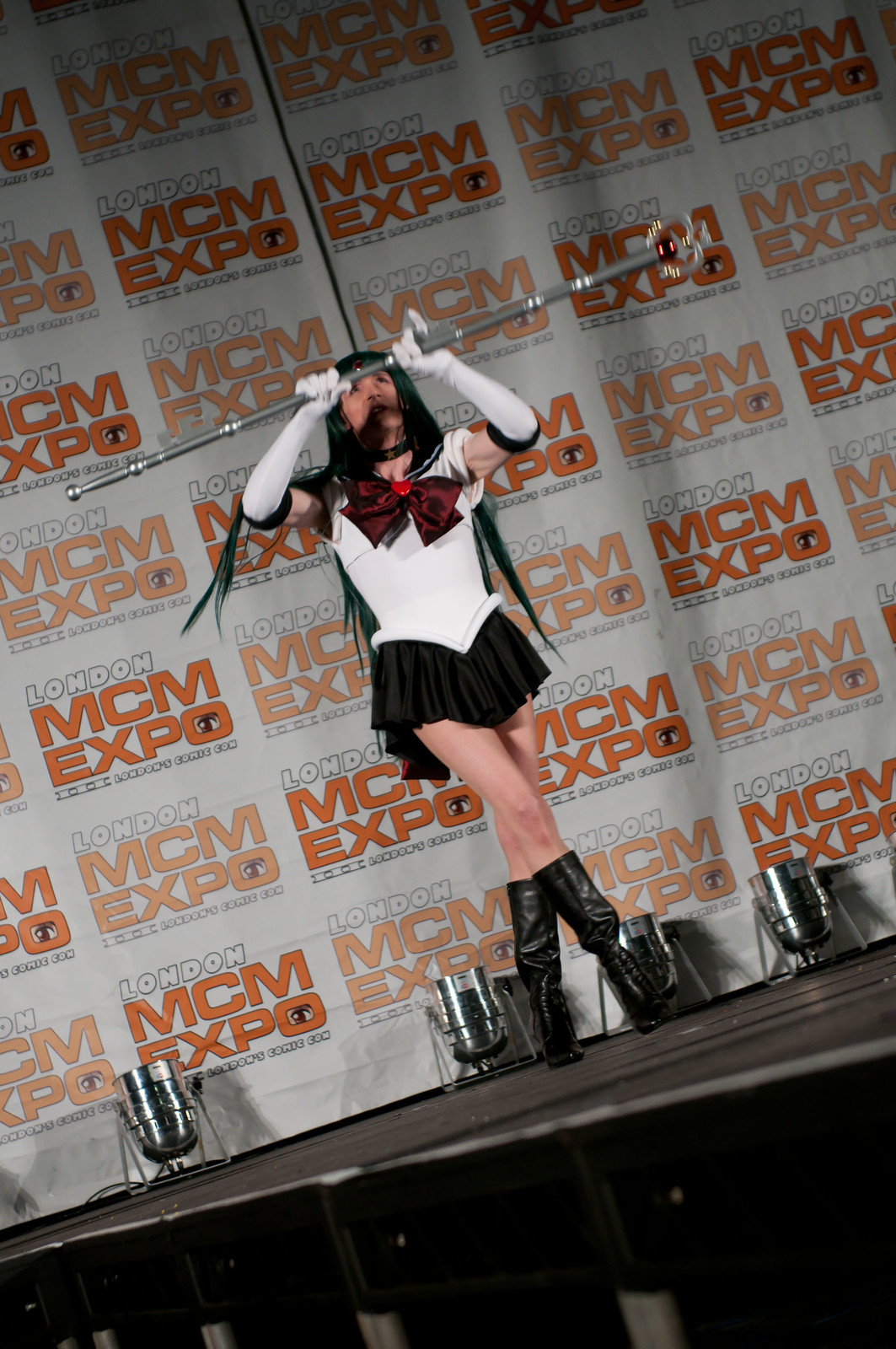The image captures a woman performing on stage, dressed in what appears to be a Sailor Moon cosplay. She is holding a long, silver staff with a shiny red, heart-shaped ornament at the end, raising it in front of her head as she looks up. Her attire includes a white top with a large dark red bow on the front, a short black skirt, and black boots that reach her upper calves. She also dons long white gloves that extend past her elbows. She has long, straight dark hair, possibly a wig, cascading down her shoulders. The background features a white banner with the text "London MCM Expo" in a repeating pattern. The perspective of the photo is from the audience's viewpoint, giving an upward angle to the scene. The moment captured shows a slight motion blur on the staff, adding dynamism to the performance she is executing.